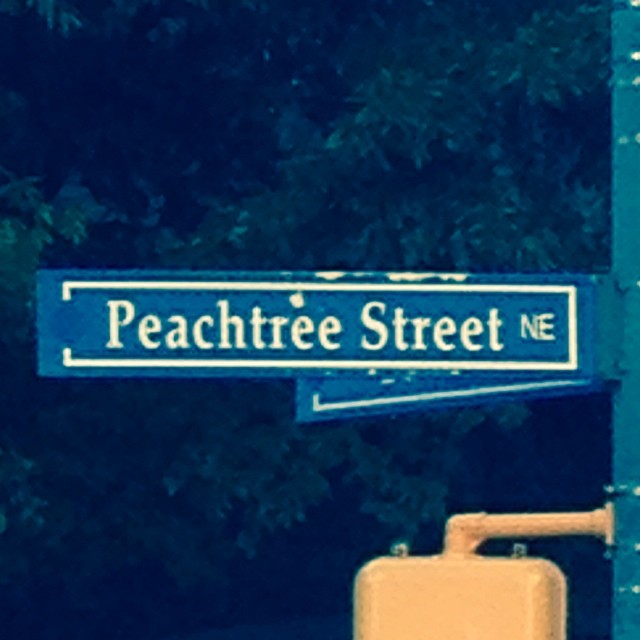This very faded color photo depicts a street scene prominently featuring a green street sign pole on the right side of the image. Attached to the pole is a green street sign with white lettering that reads "Peachtree Street N.E." The sign is positioned above a yellow traffic light system, although the traffic light isn't fully visible in the frame. To the right, the green pole is distinct against the backdrop. The large street sign and traffic light system suggest the photo was taken at a street corner. In the background, dense dark green trees and foliage dominate the scenery, indicating low light conditions, either due to an overcast weather or the photo being taken early or late in the day. On the left side of the picture, another street sign is partially visible at a perpendicular angle, though its details are obscured.